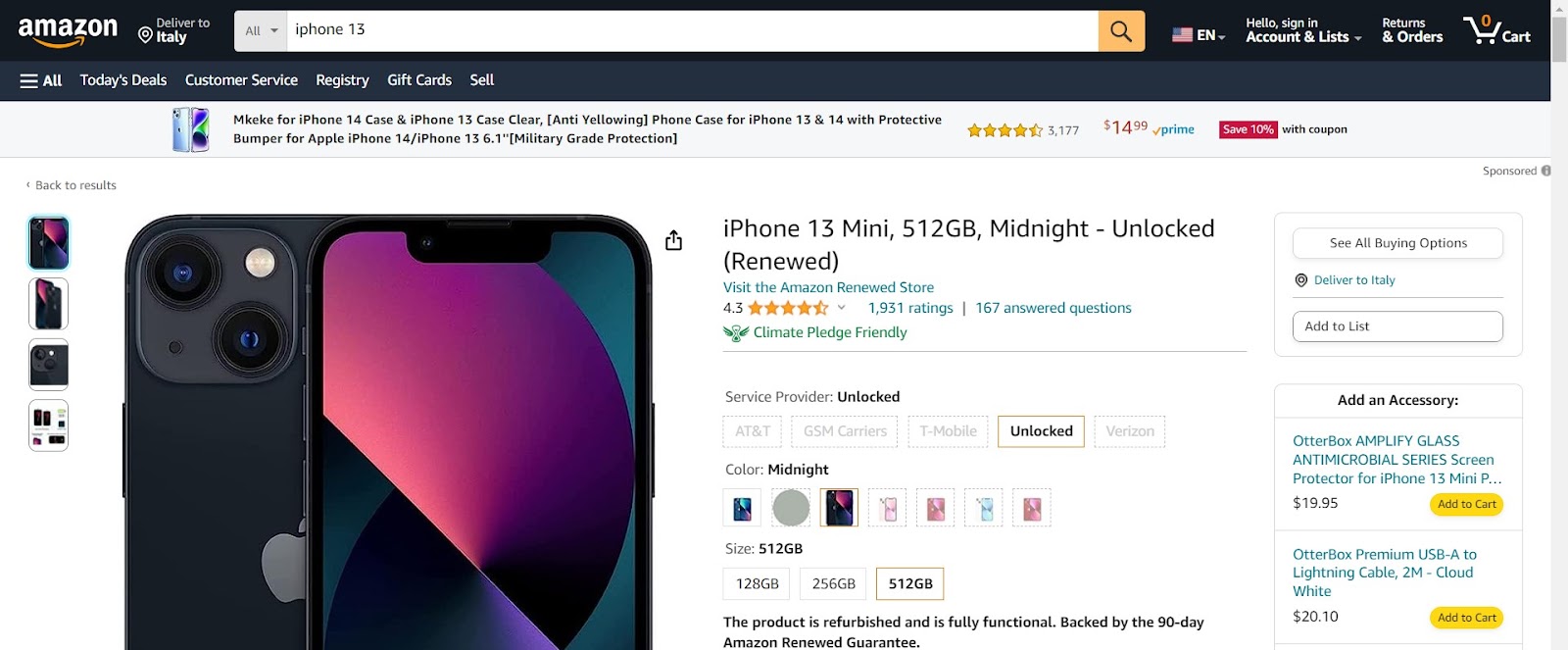The image shows an Amazon page for the "iPhone 13 Mini, 512GB, Midnight, Unlocked, Renewed." The browser displays several UI elements, including a search bar with "iPhone 13" typed in it, and options such as "Hello, Sign In," "Accounts & Lists," "English for the language (American English)," "Returns & Orders," and "0 in Cart."

The product, an iPhone 13 Mini with 512GB storage in the Midnight color, is highlighted as a renewed item, indicating it has been refurbished and is fully functional, backed by a 90-day Amazon Renewed Guarantee. The device has received a rating of 4.3 stars from 1,931 reviews and has 167 answered questions. It is labeled as "Climate Pledge Friendly" and is compatible with unlocked service providers. 

Additional buying options and accessory suggestions are provided on the right side of the page. These include options to "Add to List" and purchase compatible accessories such as the OtterBox Amplify Glass Antimicrobial Series Screen Protector for $19.95, and the OtterBox Premium USB-A to Lightning Cable (2 meters, Cloud White) for $20.10. 

The page indicates that the item can be delivered to Italy.